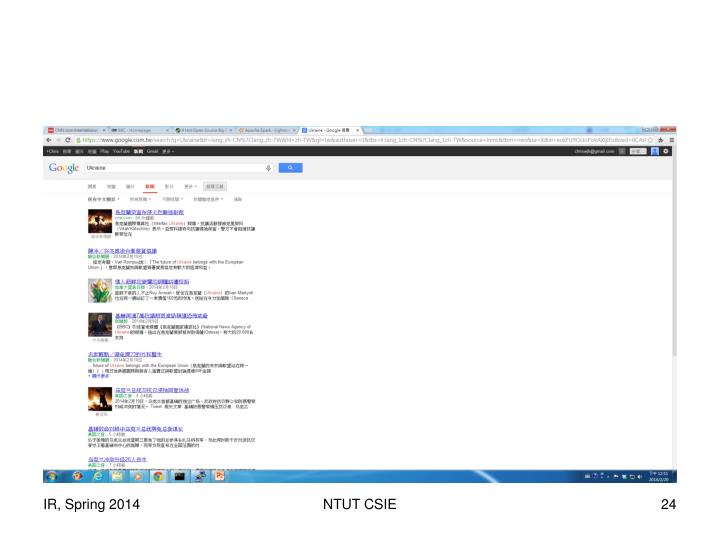The image is a low-resolution screenshot of a Google search results page displayed on a Windows computer. The screenshot captures the browser with five tabs open, where the first four tabs have a gray background and the fifth is highlighted in white. Below the tabs, there's the search bar indicating google.com, but the specific search query isn't readable. The familiar Google logo is positioned above the search box, adjacent to a blue search icon. The search results are predominantly in Chinese and each result features a picture to its left, although the finer details of these results are indistinguishable.

Along the bottom of the screen, there's a blue bar showcasing various icons including Google Chrome and Internet Explorer. Visible text includes "IR Spring 2014" and "NTUTCSI" with the number "24" appearing in the bottom right corner. The assortment of colors in the screenshot includes red, blue, white, brown, black, green, and yellow, amid the predominantly white and blue interface of the Google search page.